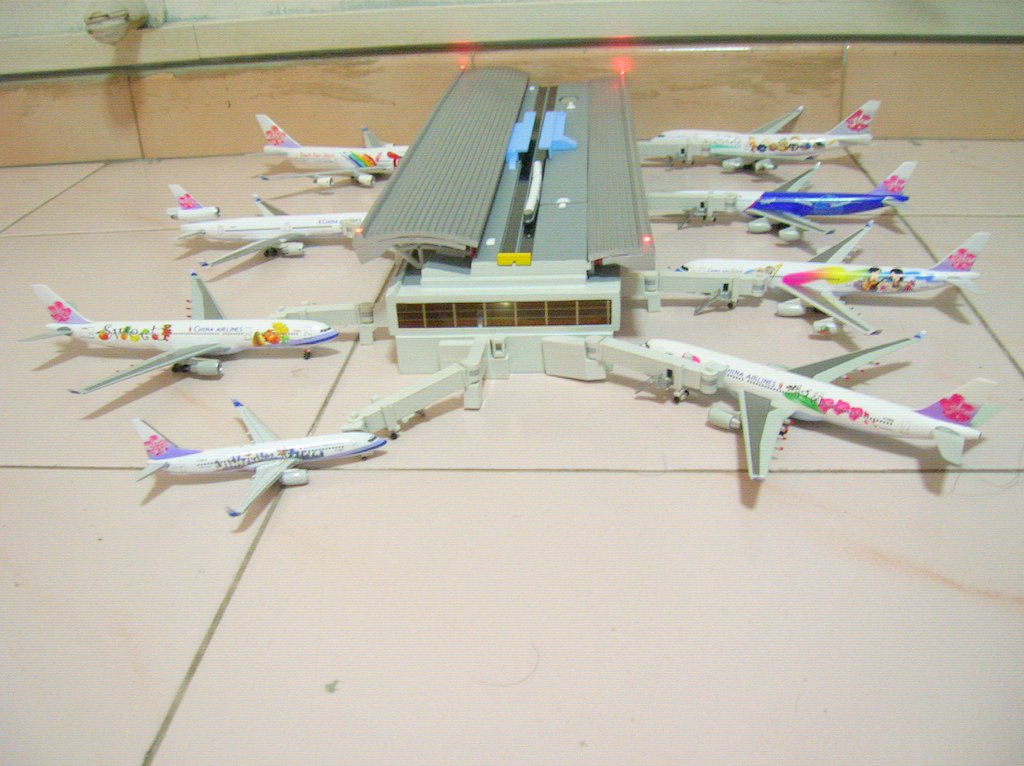This photograph showcases a small-scale model of an airport terminal, prominently displayed on a large, pale pink-tiled floor with gray grout and an off-white baseboard running along the tiles. The airport model features a modern white building with a gray roof and blue accents, likely representing air conditioning units, along with detailed white tubing resembling HVAC systems. Large windows run along the sides and ends of the terminal, allowing views of the inner layout. Surrounding the terminal are eight model passenger jets positioned at the gangways, each intricately detailed to mimic real-life airport scenes. 

The jet planes are designed with tropical themes, predominantly white with various colorful designs. On the left side, the planes are adorned with pink flowers and fruit motifs, whereas on the right side, they feature similar colors but with one plane prominently painted cobalt blue at the rear. Additional design details include a plane with two figures painted on the tail. Two more planes are positioned differently; one is smaller and tilted to the right, and another faces left with pink flower designs, adding to the realistic and lively ambiance of this airport demonstration model.